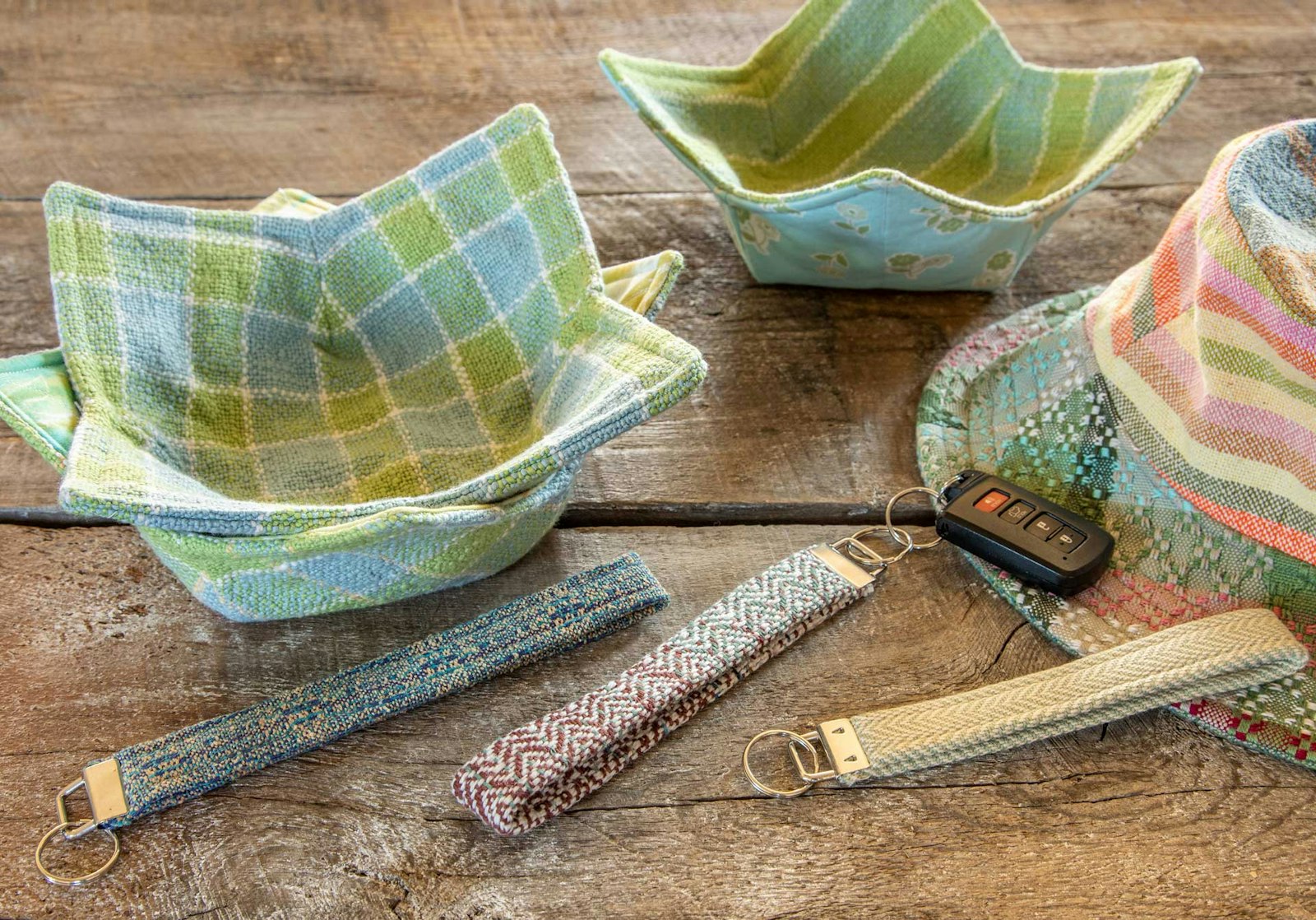The image showcases a collection of handmade fabric items artfully arranged on a rough, unfinished wooden table marked with scratches. At the center lie three distinct, colorful cloth keychains. The leftmost keychain is predominantly blue, embellished with multicolored speckles of orange and yellow. In the middle, a keychain fades from dark red into green, adorned with white zigzag patterns. The rightmost keychain stands out with an off-white hue and a tire tread design. These keychains include a metallic loop attached to the bottom, with one featuring a black key fob.

To the left, two fabric star bowls, designed with green and blue stripes and a contrasting floral exterior, add a touch of intricacy. One bowl nests within the other, while a third similar bowl sits close by. 

On the right side of the image, a multicolored woven hat with muted tones of yellow, pink, green, and specks of blue complements the scene. Its speckled brim suggests a cozy, handmade aesthetic suitable for a day at the beach. The entire composition gives off a charming, artisanal vibe, reminiscent of a well-curated Etsy shop display.